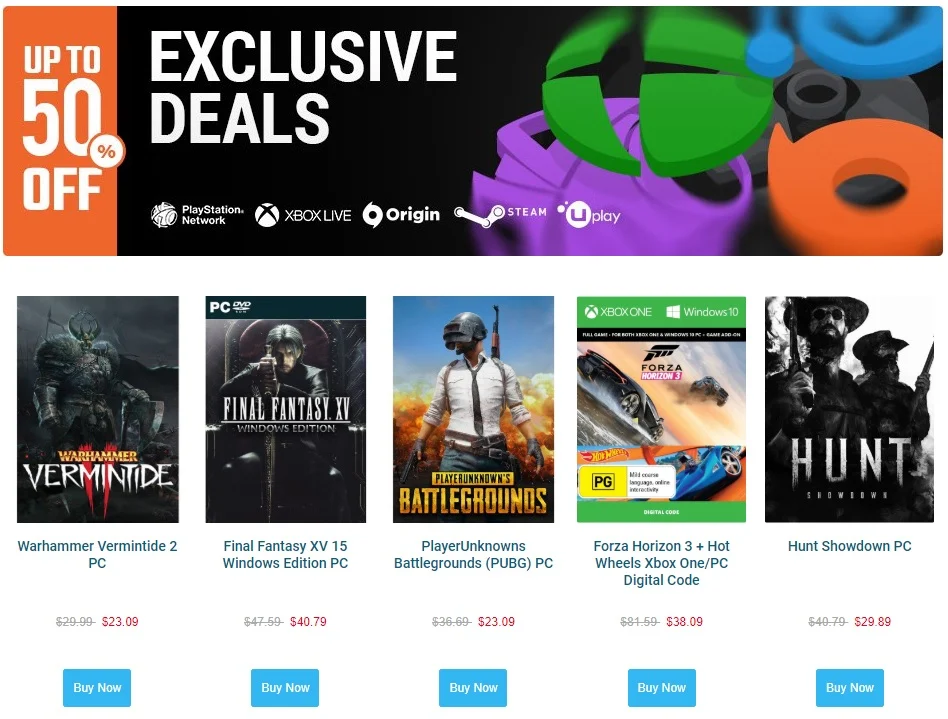The image showcases a website's main banner highlighting exclusive deals. The top of the banner prominently displays an orange section on the left side, announcing discounts of up to 50%. The central portion emphasizes the theme of "exclusive deals" and features logos from various popular gaming platforms: PlayStation Network, Xbox Live, Origin, Steam, and Uplay. The background is black, adorned with differently colored abstract shapes — green, blue, gray, orange, and purple.

Below the banner, a selection of discounted games is displayed. From left to right, the games and their discounts are:

1. **Warhammer: Vermintide 2 (PC)** - Originally priced at $29.99, now available for $23.09. A "Buy Now" button is included.
2. **Final Fantasy XV Windows Edition (PC)** - Originally priced at $47.50, now available for $40.79. A "Buy Now" button is included.
3. **PlayerUnknown's Battlegrounds (PC)** - Originally priced at $36.69, now available for $23.09. A "Buy Now" button is included.
4. **Forza Horizon 3 Plus Hot Wheels (Xbox One/PC Digital Code)** - Originally priced at $81.50, now available for $38.09. A "Buy Now" button is included.
5. **Hunt: Showdown (PC)** - Originally priced at $40.79, now available for $29.89. A "Buy Now" button is included.

The overall layout is visually engaging, directing the viewer’s attention to the substantial savings on popular gaming titles.